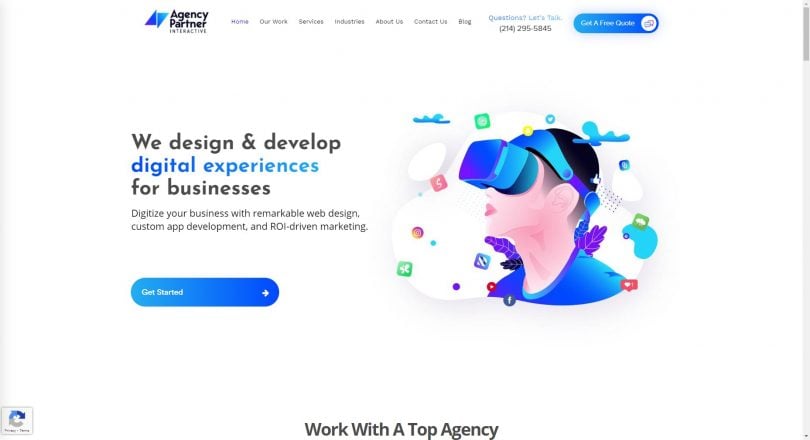The image features a screenshot of a small laptop or tablet displaying the website of a company named "Agency Partner Interactive." The website's navigation bar at the top includes links to Home, Services, Industries, About Us, Contact, and a phone number for inquiries. A prominent button labeled "Get a Free Quote" is also present.

The main tagline prominently states, "We design and develop digital experiences for business," followed by a description: "Digitize your business with remarkable web design, custom app development, and ROI-driven marketing." Below this description, there is a call-to-action button inviting users to "Get Started."

At the bottom of the webpage, text highlights the company's credibility with the phrase "Work with a top agency."

The central part of the image features an animated illustration showing a person wearing an AI mask and an accompanying headband. Surrounding the person's head are floating symbols and icons, representing various apps and digital tools, creating a cloud-like effect. These symbols emphasize the diverse digital solutions and development services offered by the agency.